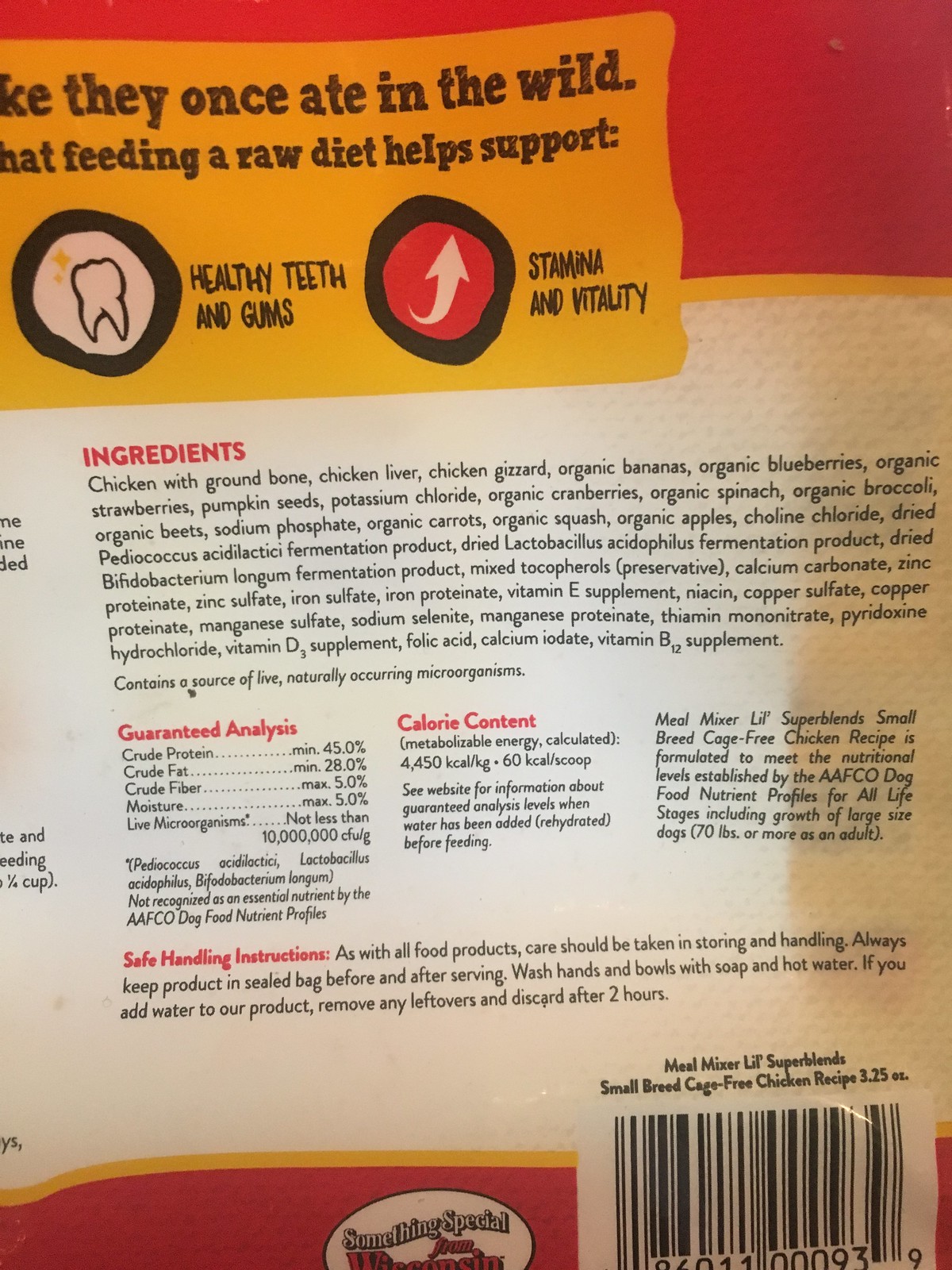This color photograph captures the back of a pet food package, showcasing a detailed and informative label. In the upper left corner, a prominently positioned box contains advertising text highlighting the product's features. This pet food aligns with a Roth diet type, emphasizing dental health with a small illustration of a tooth indicating benefits for healthy teeth and gums.

To the right, an eye-catching red circle encloses an arrow with the words "stamina and vitality," emphasizing the energetic benefits of the food. Below this, an extensive and meticulously detailed list enumerates the ingredients contained within the package, followed by a comprehensive nutritional analysis and a calorie count.

Further down, the brand name appears alongside a thorough product description, succeeded by handling instructions and safety information, written in a smaller font. Headers throughout the label are styled in bold red lettering, contrasted with black text beneath for the main content.

Positioned in the bottom right corner is a barcode, next to which a small additional logo for the product is placed. The image focuses entirely on the label, without capturing any parts of the package’s top, bottom, left, or right sides, providing a clear view of the information presented.